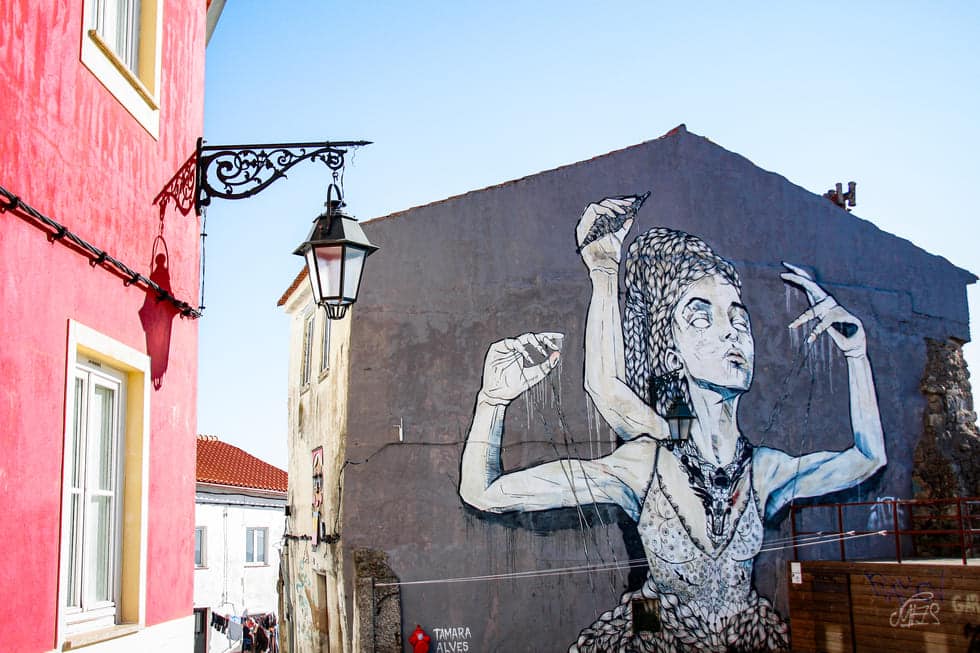This outdoor photograph captures a sunny day with a clear, blue sky, showcasing several buildings. A dominant red building spans the left side of the image, identified by its two white-trimmed windows and a black wall sconce extending out, casting a shadow. Adjacent to this, towards the center, stands a striking mural painted on the dark gray side of a building, encompassing most of the photograph. The mural, attributed to the artist Tamara Alves, features a woman with three arms. Her two primary arms are raised in a V shape, while a third arm extends from her back, gripping an object that appears to be tapered at both ends. The woman is depicted in a black dress with a feathery white and tan skirt, a camisole top, and a distinctive turban with a black or brown pattern. She has white eyes, suggesting blindness or a spiritual aura, long braids, and longer nails. The mural details also include a black necklace and bracelets. To the left of this mural building is a pinkish-red building, marked by a jutting lantern and its shadow. Further in the background, a white house with a red roof is visible, coupled with a glimpse of laundry hanging in an alleyway.